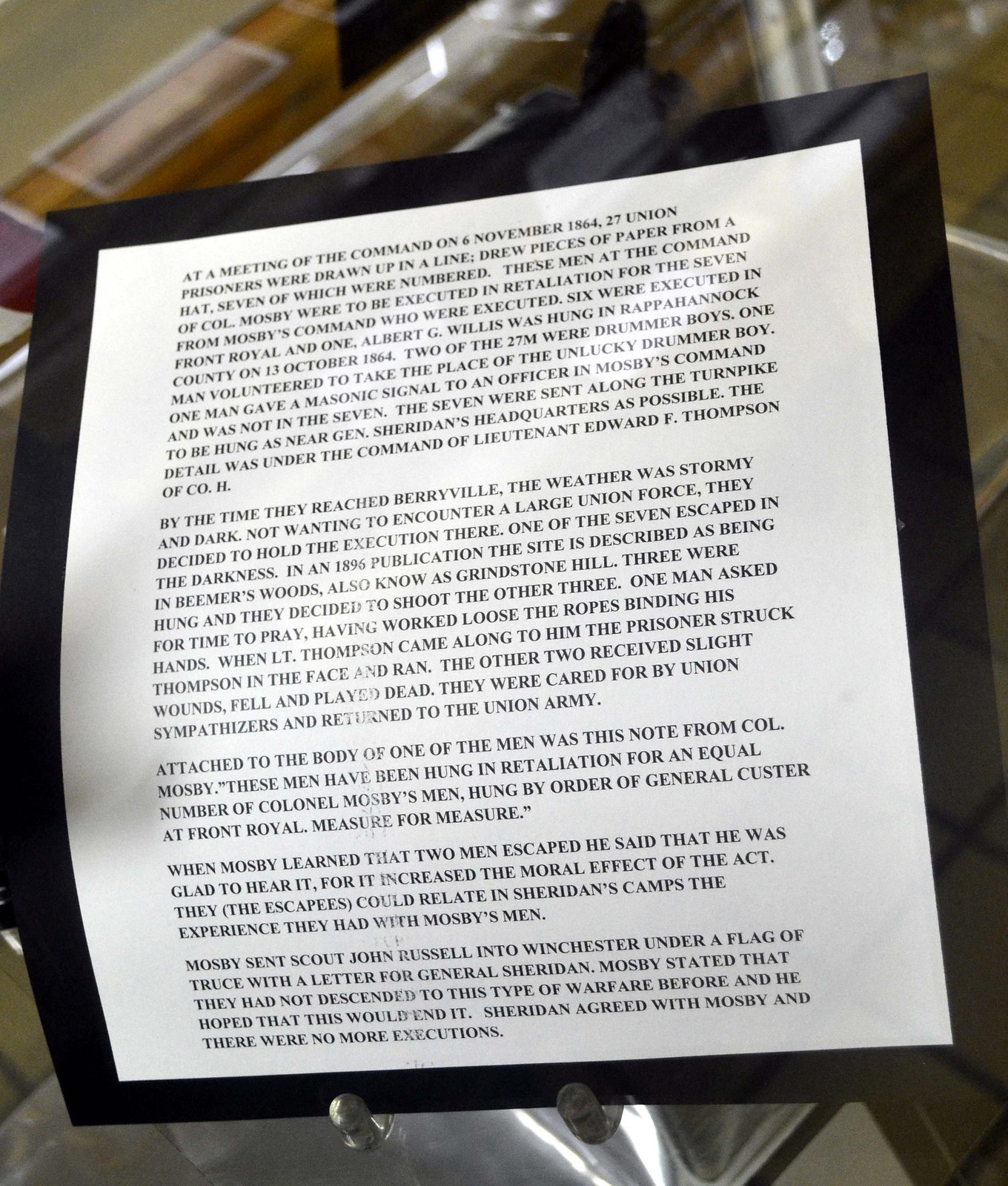This photograph depicts a historical plaque on a white piece of paper with black, all-caps text, framed by a black border and slightly curled. The text provides a detailed account of a retaliatory execution during the American Civil War. It reads: "At a meeting of the command on 6 November 1864, 27 Union prisoners were drawn up in a line and drew pieces of paper from a hat, seven of which were numbered. These men, at the command of Colonel Mosby, were to be executed in retaliation for seven of Mosby's men who had been executed by order of General Custer at Front Royal. Six men were executed in Front Royal, while one, Albert G. Willis, was hung in Rappanoag County on 13 October 1864. Among the 27 prisoners were two drummer boys; one man volunteered to take the place of a drummer boy, and another was spared after giving a Masonic signal. The seven condemned men were sent along the turnpike to be hung near General Sheridan's headquarters. The executions were carried out under the command of Lieutenant Edward F. Thompson of CO.H. During a stormy night near Beemore Swords, also known as Grindstone Hill, the execution was attempted: three were hanged, three were shot, and one managed to escape. Attached to the body of one of the executed men was a note from Colonel Mosby reading, 'These men have been hung in retaliation for an equal number of Colonel Mosby's men hung by order of General Custer at Front Royal, measure for measure.' Mosby later expressed relief that two men had escaped, hoping the story would spread the harsh reality of war and deter future such actions. Following this, Mosby sent Scout John Russell under a flag of truce to deliver a letter to General Sheridan, expressing a desire to end this type of warfare. Sheridan agreed, and no further executions occurred." In the background, a glass table is slightly visible, adding to the solemn atmosphere of this poignant memorial.